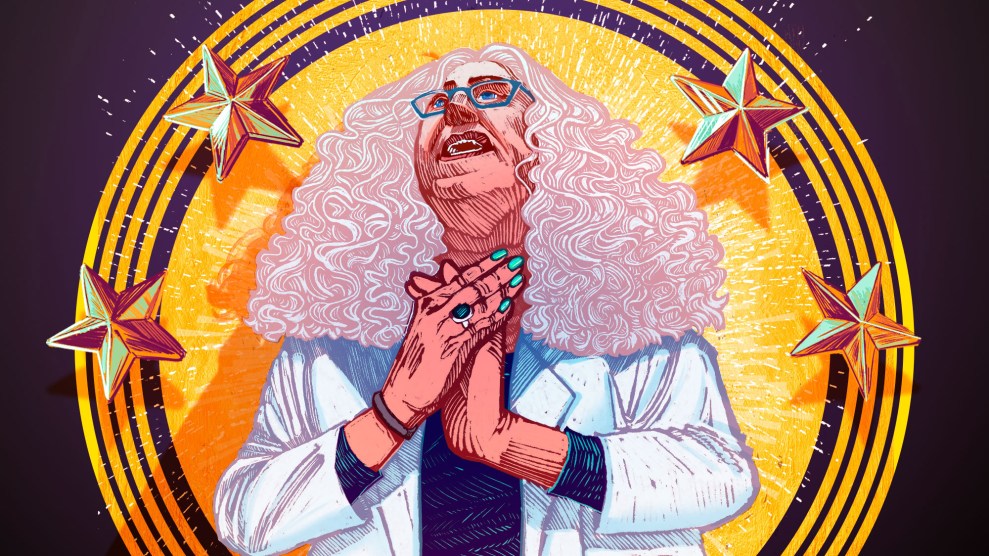This detailed digital illustration features a caricature of an older woman with distinctive long, curly white hair that is intricately outlined in pink. She dons blue-framed glasses and has pronounced facial features, including a large nose and a big mouth. Her neck is depicted with several ruffled layers, adding texture to her caricatured appearance. The woman wears a white jacket over a blue shirt, and her turquoise-painted fingernails are prominent as she clasps her hands in front of her. Adding to her intricate attire is a turquoise ring on her right hand. She stands against a vibrant backdrop dominated by a large, solid orangey-gold circle at the center, surrounded by four concentric rings of the same color. Four five-pointed gold stars accentuate the edges of this central design. Further enhancing the background is a vast black space adorned with glittering stars, creating the impression of celestial light extending outward.